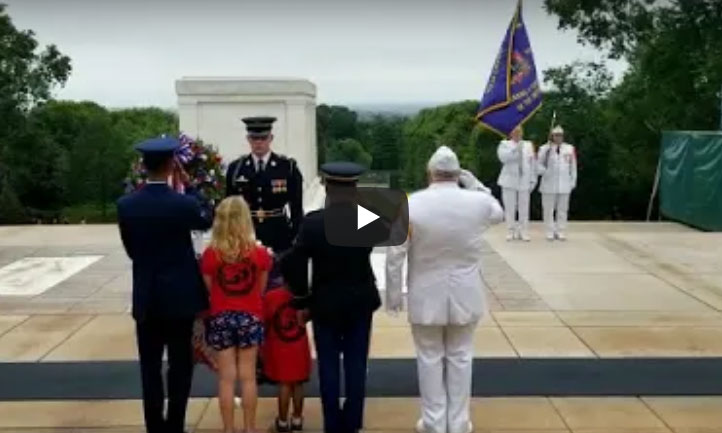This image, appearing to be a paused video clip, shows a solemn military ceremony, possibly a memorial or a service at the Tomb of the Unknown Soldier. Central to the image is a play button indicative of a video. In the scene, a man in a military uniform holds a wreath while being saluted by five individuals: two small children in red tops and three adults, all in military attire—one in blue, another in dark blue or black, and the third in white. To the right, two men dressed in white, one holding a rifle and the other a large blue flag, stand solemnly. The ceremony takes place outdoors under a cloudy sky with green trees in the background.